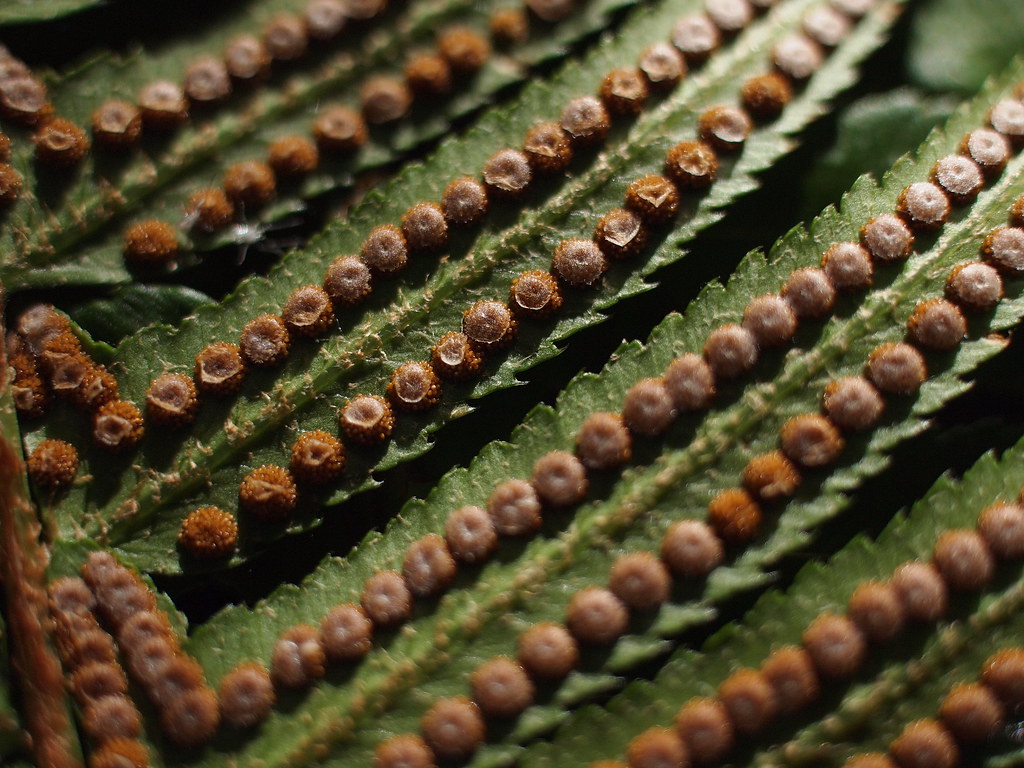The image features a highly detailed and repeating design of green pods, possibly resembling aloe vera or ferns. These pods have long, pointed ends and are lined with small, sharp spikes along their sides. Uniform rows of small, brown, seed-like circles run the entire length of these green structures, and additional clusters of these brown circles are visible on the left side of the image. The composition showcases only green and brown hues, contributing to its soothing and visually appealing uniformity. While it might resemble something natural, the precision and order in the pattern could also suggest that the image was generated or enhanced by AI. The overall effect is a captivating and harmonious display of shapes and colors.